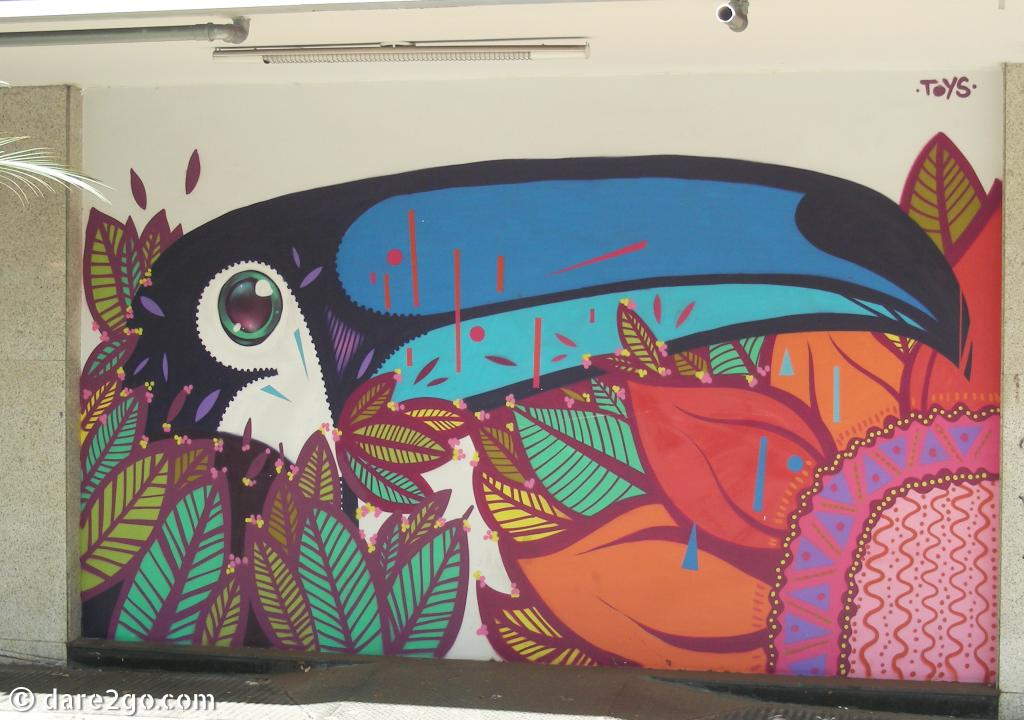This image showcases a large, tastefully painted mural on an outdoor wall with a cream-colored background. Dominating the mural is a vibrantly colored toucan, its impressive beak featuring multiple shades of blue, from dark to light sea blue, and a hint of teal. The toucan's eye captivates with its green outer layer and a purplish-black center. Surrounding the toucan are lush, intricately designed leaves in varying hues of green, some trimmed with a touch of purple, creating a lively and natural feel.

The scene is further embellished with an array of flowers, including yellow and red tulips, and a striking pink and purple flower with orange and red petals. In the mural's top right corner, the word "TOYS" is boldly displayed in capital letters and purple color, adding an element of playful text.

At the bottom left-hand corner, there is a white "C" enclosed in a circle along with the text "dare2go.com," indicating the artwork's credit. To the bottom right, a decorative section features a sketch pattern with purple triangles interspersed with red streamer-like swirls against a pink background, lending a whimsical touch to the mural's overall vibrant and fun composition.